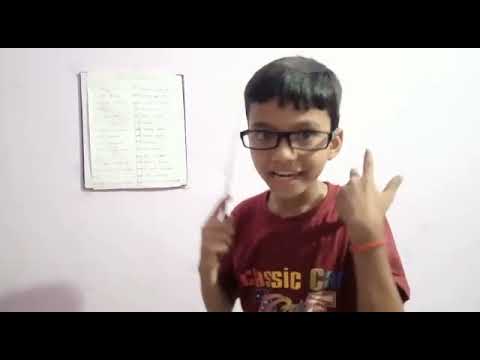The photograph features a young boy with a tan or Middle Eastern complexion, positioned on the right side of the image. He has short, dark black hair and wears slightly oversized black-framed glasses. The boy is dressed in a brownish-red short-sleeved t-shirt with the word "classic" and a cartoon character printed on it. He is posing as if he is instructing or explaining something, with his right hand holding a ruler and his left hand raised, thumb and index finger pointed upwards. His face is illuminated by a light source from the right, casting a glare on his glasses and highlighting his open mouth and visible teeth as he appears to be speaking. 

The background is a white wall, and in the top left corner, there is a yellow sheet of paper with blue or black text, possibly a checklist with two columns and small squares. A small shadow is visible in the lower left corner of the image.